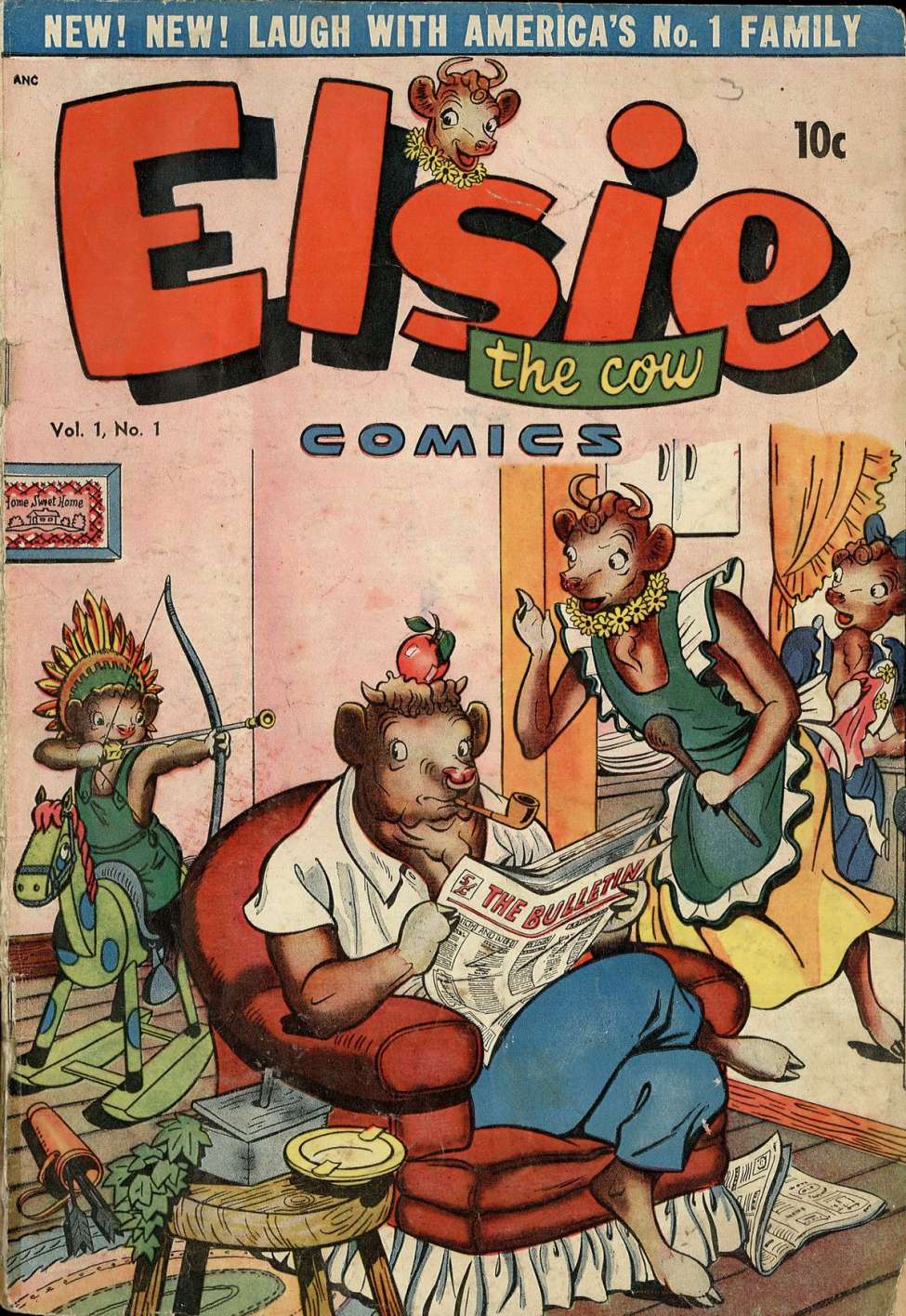This image is a scan of a vintage comic book titled "Elsie the Cow Comics," Volume 1, Number 1, which originally sold for 10 cents. The comic book features a detailed, hand-drawn cover with pronounced shadows. At the top, a blue banner reads, "New New Laugh with America's Number One Family," and below it, the title "Elsie the Cow Comics" is spelled out in large, red cursive letters outlined in black. A small illustration of Elsie the Cow’s head appears above the title, and the number "10 cents" is displayed to the right.

The main illustration showcases an anthropomorphic cow family in a domestic scene. Elsie the Cow, wearing a green apron over a yellow dress, is seen on the right, seemingly scolding a child who is riding a wooden horse and playing with a toy bow and arrow. The child, adorned with a feathered headpiece, appears to be aiming at an apple placed on the head of the father cow, who sits in a red armchair, dressed in a white shirt and blue pants, reading a newspaper titled "The Bulletin" and smoking a pipe. In the background, a female cow, possibly a daughter, is dressed in blue and appears to be engaged in kitchen chores, somewhat behind Elsie. The detailed scene captures a lively and humorous moment within the cow family, reflecting the playful and whimsical nature of the comic.